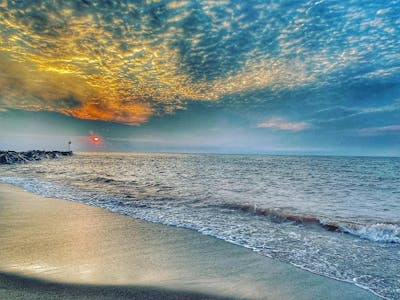The image captures a serene beach scene at either dawn or dusk, featuring the dramatic transition of the sky as the sun, a white and red orb, hovers close to the horizon. The sun-kissed clouds display a rich gradient, shifting from deep red-orange near the sun to bright yellow, with bluish-gray and darker clouds further away. The expansive sky meets a restless ocean or large lake, which has small waves lapping up onto the shore. The wet sand, exhibiting a grayish-bluish hue with patches of white, stretches from the bottom right corner to the bottom left corner of the image. On the left, a rock pier or jetty juts out into the water, adding a striking element to the scenic composition.